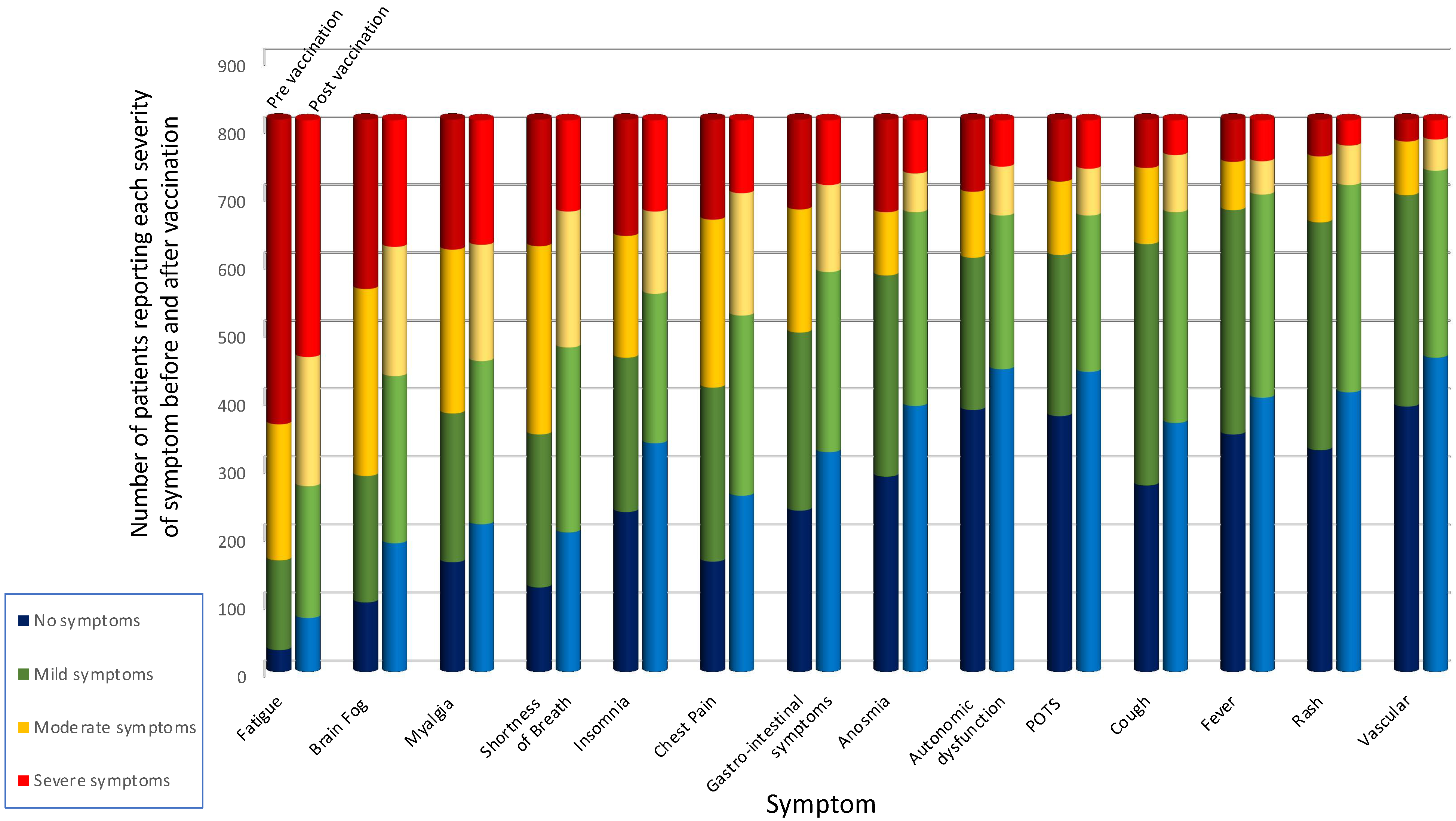This image depicts a detailed bar chart comparing the number of patients reporting various severities of symptoms before and after vaccination. Vertically, the y-axis ranges from 0 to 900, indicating the number of patients. On the horizontal x-axis, a wide array of symptoms are listed, including fatigue, brain fog, myalgia, shortness of breath, insomnia, chest pain, gastrointestinal symptoms, anosmia, autonomic dysfunction, POTS, cough, fever, rash, and vascular issues.

Each symptom is represented by two sets of bars, showcasing symptom severity with color-coded segments: blue for no symptoms, green for mild symptoms, yellow for moderate symptoms, and red for severe symptoms. The legend clarifies these colors and helps identify the severity levels. Notably, fatigue exhibits the highest severity, while vascular issues remain the least severe. Conversely, anosmia, POTS, and cough are among the symptoms most frequently reported as having no symptoms after vaccination.